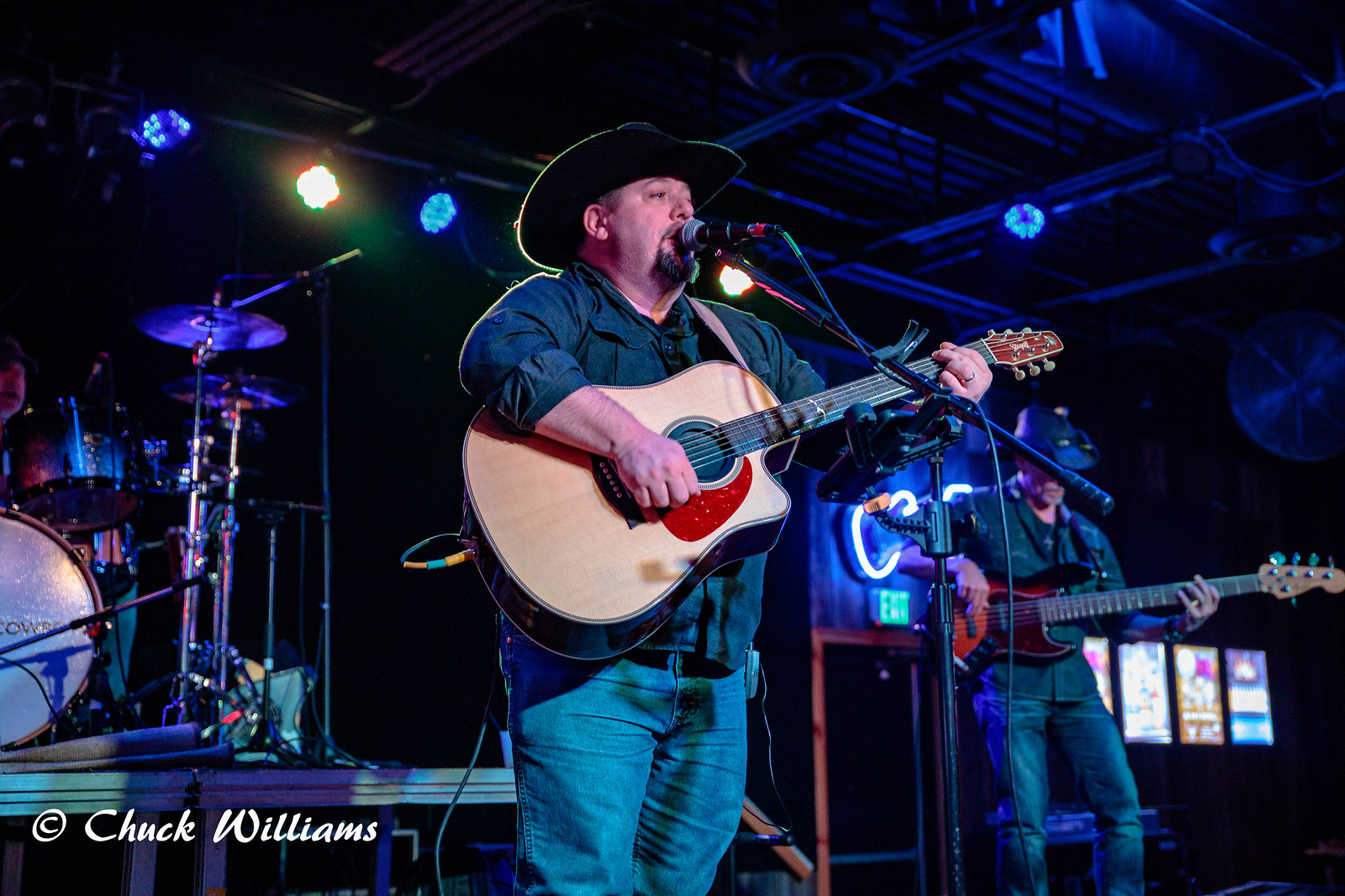This photograph, captured by Chuck Williams and marked with his copyright at the bottom right, showcases a country music band performing inside an industrial-style venue, perhaps a nightclub or bar. The focal point is the main singer, a larger gentleman in a black cowboy hat, blue jeans, and a blue jean jacket shirt, strumming an acoustic guitar and singing into a microphone. To the right stands an older bass guitarist, dressed similarly in blue jeans and a long-sleeved blue jean shirt, also wearing a cowboy hat. Behind the main singer, partially visible to the left, is the drummer amidst his drum set. The backdrop features industrial elements with lights on the top left and right, and a neon light drawing of a guitar on the wall on the right, adding to the vibrant atmosphere.